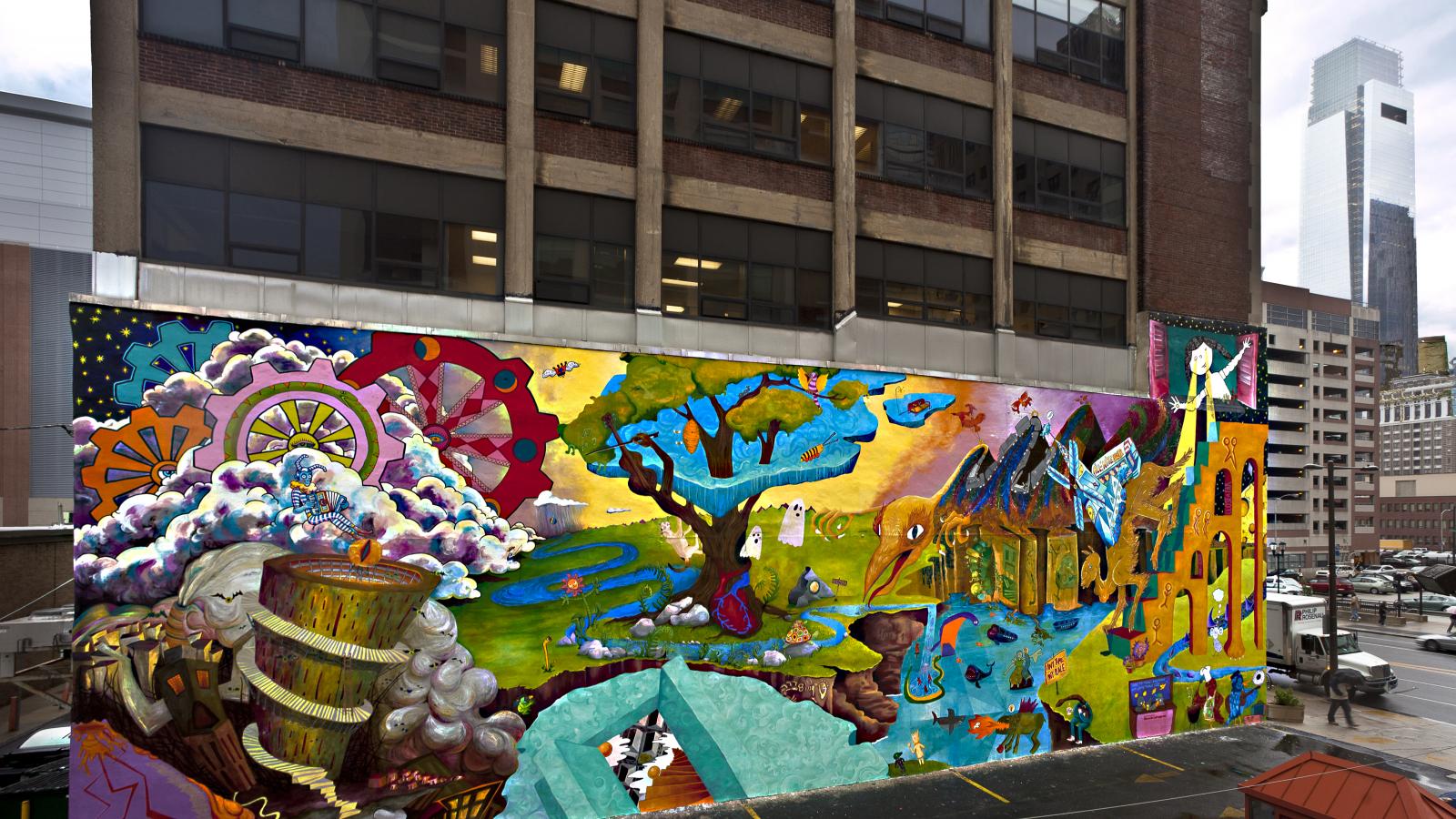In this vibrant cityscape, an office building showcases a large, hand-painted mural that dominates its lower half. The building itself is composed of brown brick with mini glass windows and faces a bustling street to the right. Surrounding the mural, other buildings with numerous windows provide an urban backdrop, including a parking garage and a sleek, silver mini-skyscraper featuring a large rectangular black window near its top. The sky above is overcast, adding a dramatic tone to the scene.

The mural is an imaginative, fantasy wonderland created with an eclectic mix of colors and styles. On its left side, vibrant gears and cogs in shades of orange, pink, red, yellow, purple, and maroon are intertwined with clouds or steam. The centerpiece of the mural is a giant tree with a lush green canopy, surrounded by ghostly blue matter and floating greenery. Beneath the tree, a stream winds through the scene, featuring a large bird's head drinking from it. 

Other elements include deconstructed buildings—formed of just windows and doors without walls—creating an ethereal, surreal environment. Little strange creatures, some resembling dinosaurs or bizarre birds with wings and claws, populate the ground near small ponds and streams. On the upper right of the mural, a person appears to be climbing or reaching out towards the intricate structures. The mural blends bright, muted, and cartoonish styles to create a dynamic and whimsical tableau that captivates the viewer's imagination.